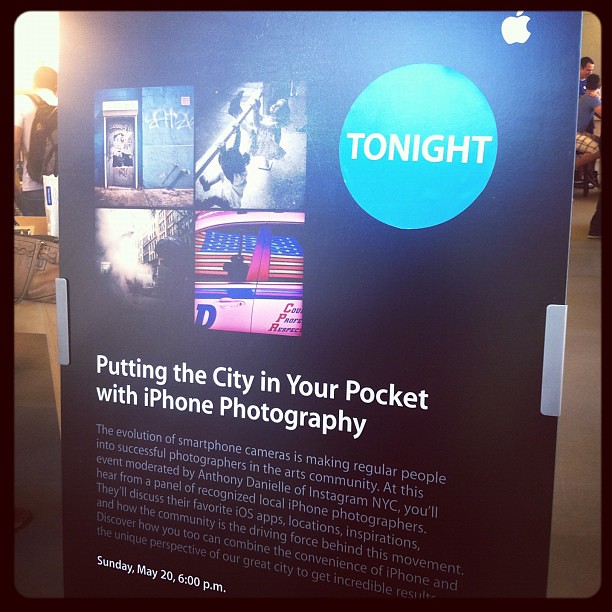This image showcases a promotional sign for an event set to take place on Sunday, May 20th at 6 p.m. The black background of the sign is prominently contrasted by white text, making the details clearly visible. At the top right-hand corner, the iconic Apple logo is displayed in white. The key phrase "Putting the City in Your Pocket with iPhone Photography" stands out, emphasizing the event's focus. 

The word "Tonight" is highlighted within a blue circle also positioned at the top right. The sign features four photographs displayed on the left side: one of a car, another in black and white with people, one of a building, and one of a staircase, showcasing the impressive capabilities of the iPhone's camera. Additionally, a detailed paragraph explains the event: smartphone cameras are empowering everyday people to become accomplished photographers. The session will include discussions led by Anthony Daniel of Instagram NYC and a panel of noted local iPhone photographers, covering topics like favorite iOS apps, inspirational locations, and the impact of community. 

Beyond the sign, the background reveals people milling about, suggesting that the image was likely taken at the event location, possibly an Apple store, convention center, or meeting hall.